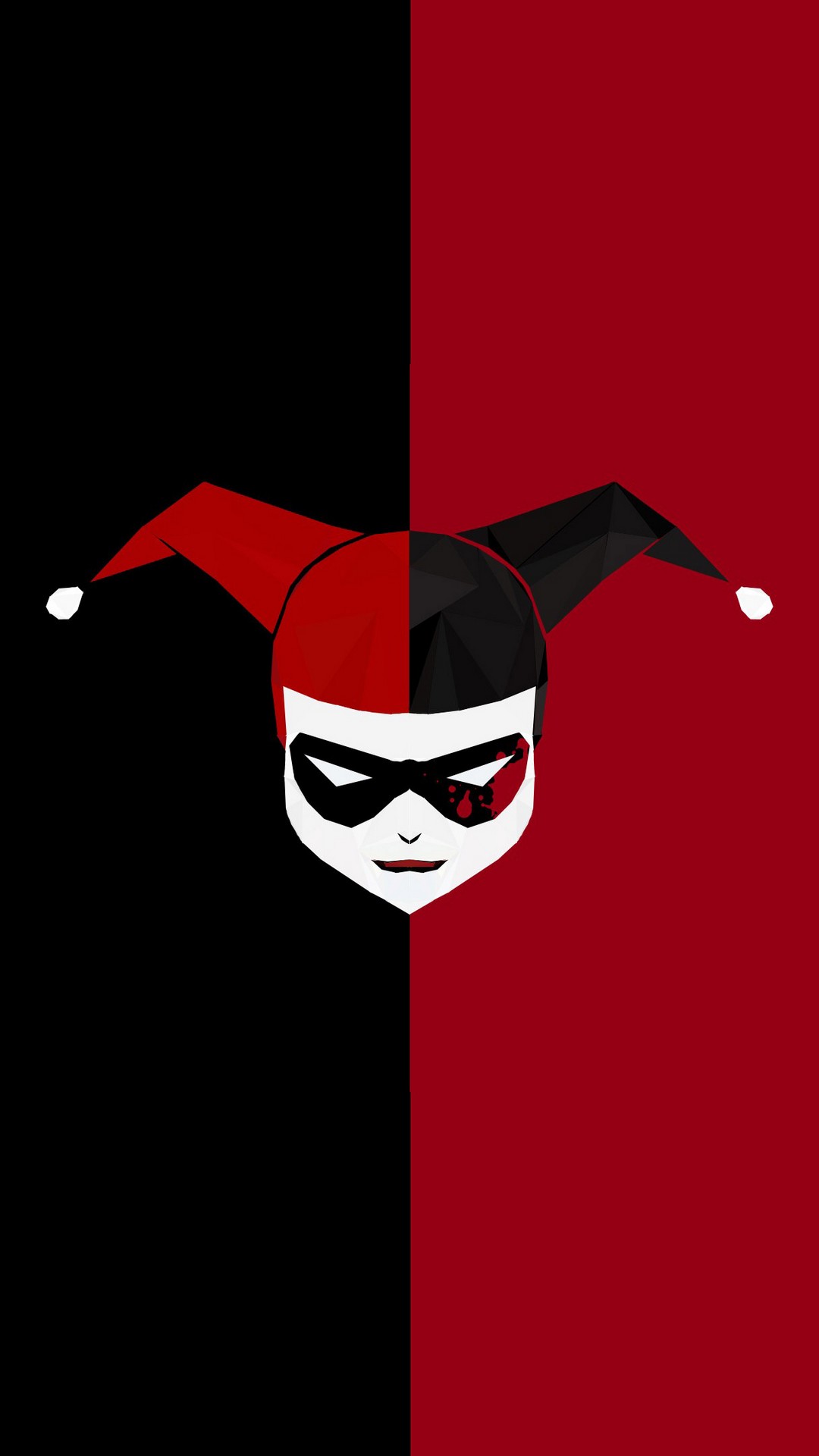The image depicts a drawn face that merges the iconic elements of Harley Quinn and the Joker, resembling the type of Joker you'd see on a deck of cards. The face is notably characterized by red lips, a pointed chin suggesting a more feminine appearance, and a mask over the eyes—mostly black with a red splotch, evocative of a blood stain. The jester hat is split into two halves: the left side is red with a white tip, and the right side is black with a white tip, perfectly complementing the evenly divided background, which is black on the left and red on the right. The mask obscures the eyes, and the expression appears neutral, with slightly pursed lips and an open mouth, though the overall impression of the facial expression is ambiguous due to the mask. The background's stark divide in color heightens the contrast and symmetry of the face and hat, with the entire composition centered precisely within the frame, creating a visually striking and balanced image.